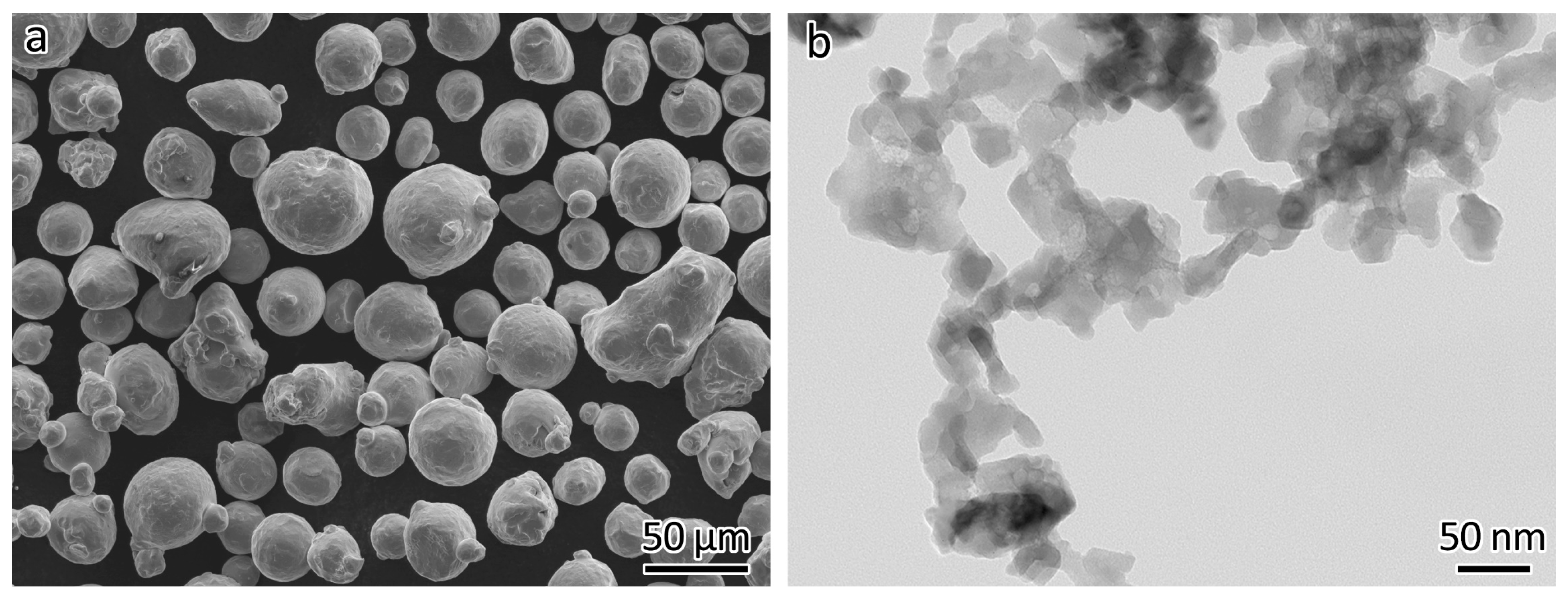The image consists of two adjacent, equal-sized photographs separated by a thin white line. The left photograph, labeled "A" with a big, black lowercase letter in the top left corner, showcases a solid black background filled with various spherical gray blobs. These blobs, which range in size and slightly differ in shape—some more oval than round—appear to be floating and closely clumped with small gaps between them. Notably, this image includes the annotation "50 UM" in the bottom right corner. The right photograph, marked "B" with a lowercase letter in its top left corner, presents a gray background with gray blobs concentrated in the center. Unlike the left, these blobs blend more seamlessly into the background, resembling a paint splatter or watercolor effect, without distinct borders. This image is annotated "50 NM" in the bottom right corner. Both photographs are in black and white and appear to capture a microscopic view of cells or microbes, highlighting their varied structures and formations.